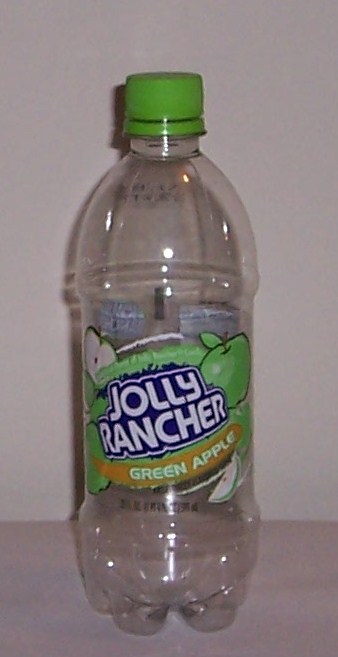The photograph showcases an empty plastic bottle of Jolly Rancher Green Apple soda. The bottle is primarily composed of transparent plastic, allowing for a clear view of its contents—or in this case, the lack thereof. The brand name, "Jolly Rancher," is prominently displayed in bold white text with a blue border at the center of the label. Below this, the flavor designation "Green Apple" is emblazoned in a stylized font, featuring a distinct swooping green graphic. To the right of the text are two vivid illustrations: one of a whole green apple and another depicting a halved apple, complete with visible seeds and a stem. Adding a pop of color, the bottle is capped with a bright green lid. Resting against a minimalist backdrop, the bottle is positioned on a white table with a plain white wall in the background, making for an uncluttered and straightforward image.